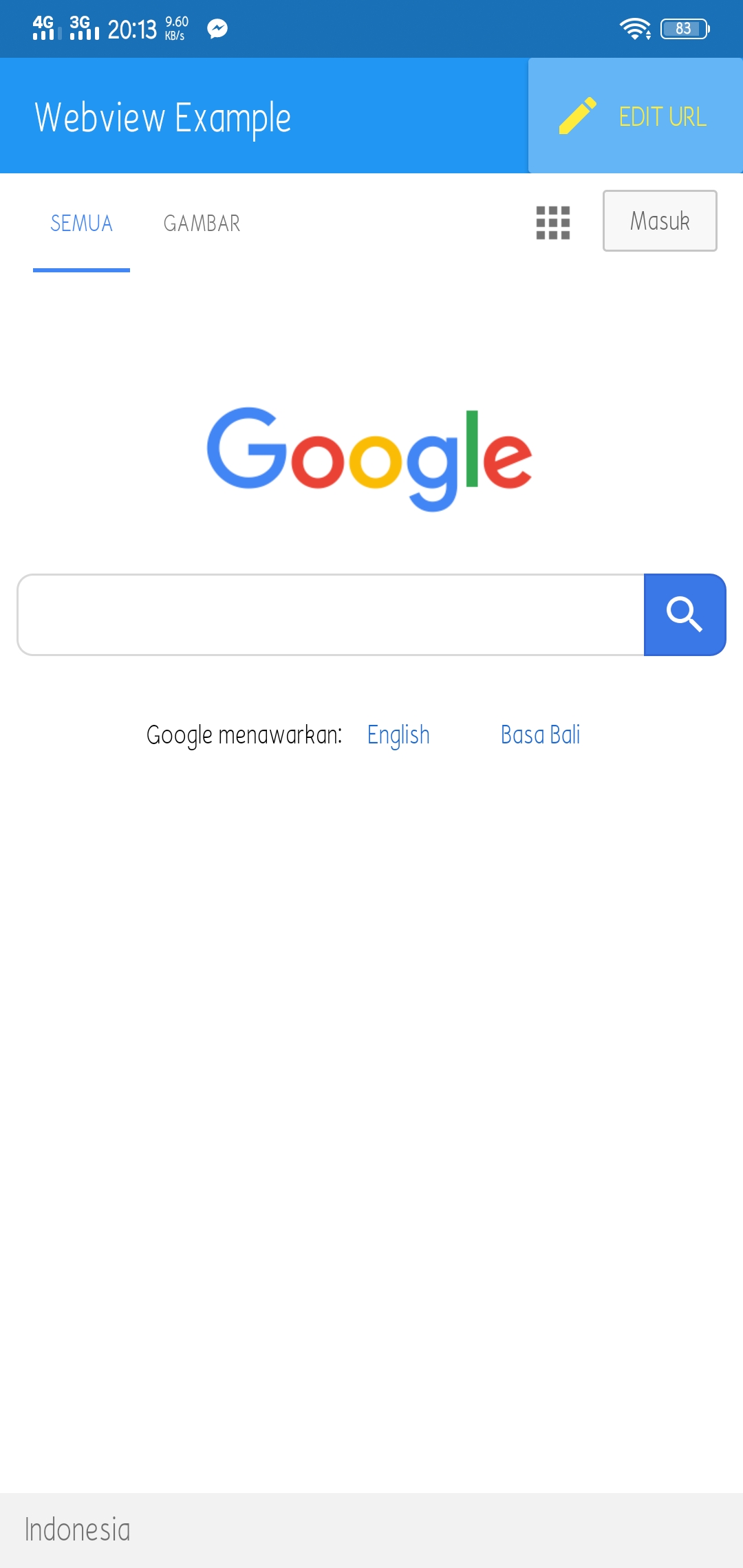The image depicts the Google homepage on a mobile phone screen. At the top left, connectivity icons display "4G" and "3G," alongside the time, which reads "20:13." To the right of the time icons, there is a messaging icon, a Wi-Fi symbol, and a battery indicator showing 63% charge, all set against a blue background.

Directly below, there is a URL bar featuring a website example with a yellow pencil icon next to it labeled "Edit URL." Beneath the URL bar are two labeled tabs: "SEMUA," which is highlighted, and "GAMBAR," indicating a tab switch option.

Central to the image is the prominent "Google" logo with a search bar placed below it. Within the search bar, on the right side, there's a blue square icon housing a magnifying glass, denoting the search function. Below the search bar, the text "Google" is repeated alongside words such as "MENAWORKON," "English," and "BASABDI,” suggesting language settings. 

The entire background of the page is white, while the very bottom left corner features a gray background with the word "Indonesia" written on it, indicating the location setting of the Google search.